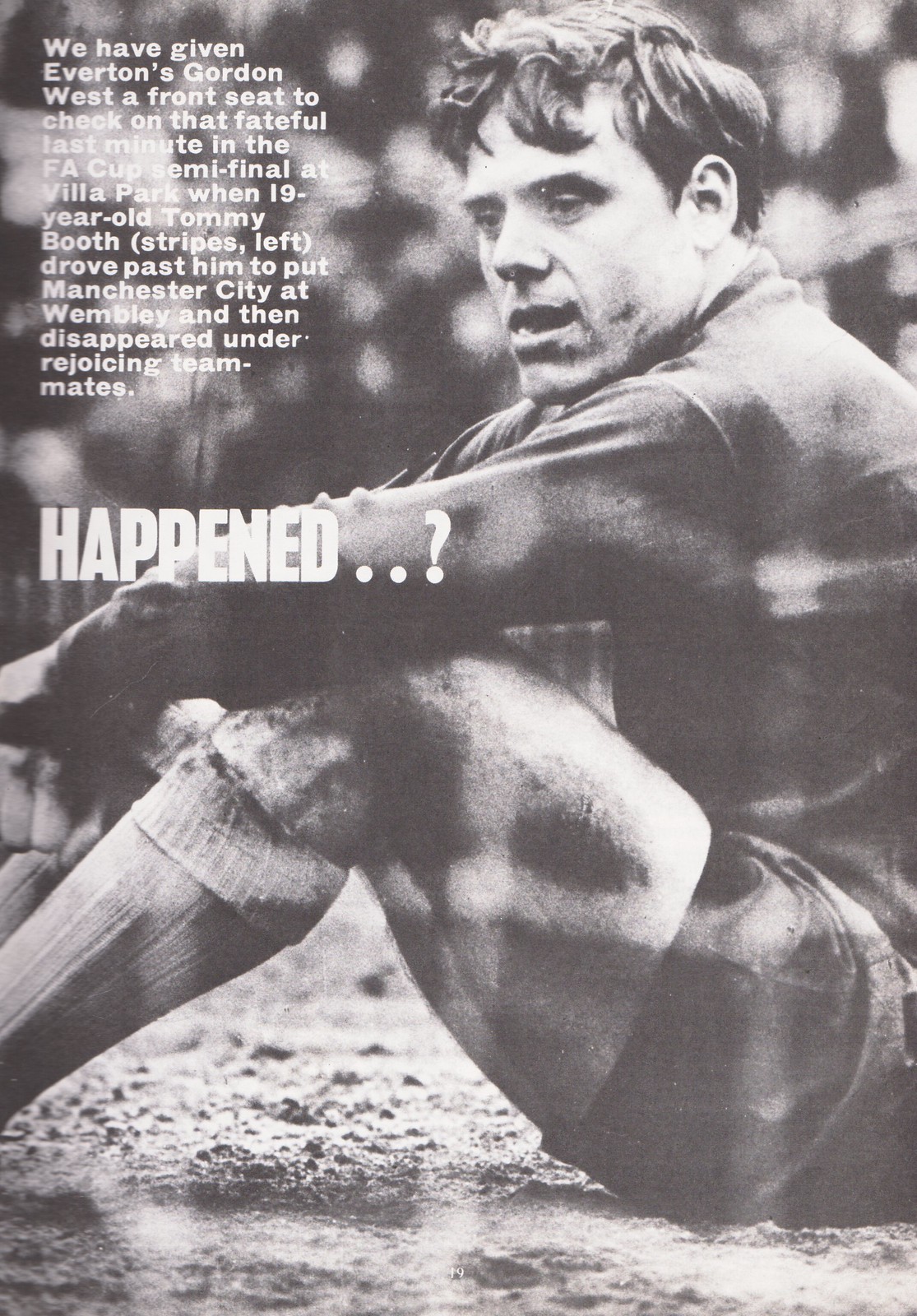The image appears to be the black-and-white front cover of a sports magazine or book. Dominating the center is a man, Everton's Gordon West, sitting in the mud with his hands resting above his knees, embodying a look of disappointment. He has short dark hair, and his mouth is slightly open as he gazes forward and to his left. He is wearing a dark shirt paired with shorts and light-colored socks, folded over at the top. The backdrop hints at a crowd of people, adding to a sense of a pivotal moment captured in time. In the top left corner, white text reads: "We have given Everton's Gordon West a front seat to check on that fateful last minute in the FA Cup semi-final at Villa Park when 19-year-old Tommy Booth, stripes left, drove past him to put Manchester City at Wembley and then disappeared under rejoicing teammates." Below that, larger text simply asks, "What happened?" conveying a sense of mystery and drama surrounding the event.